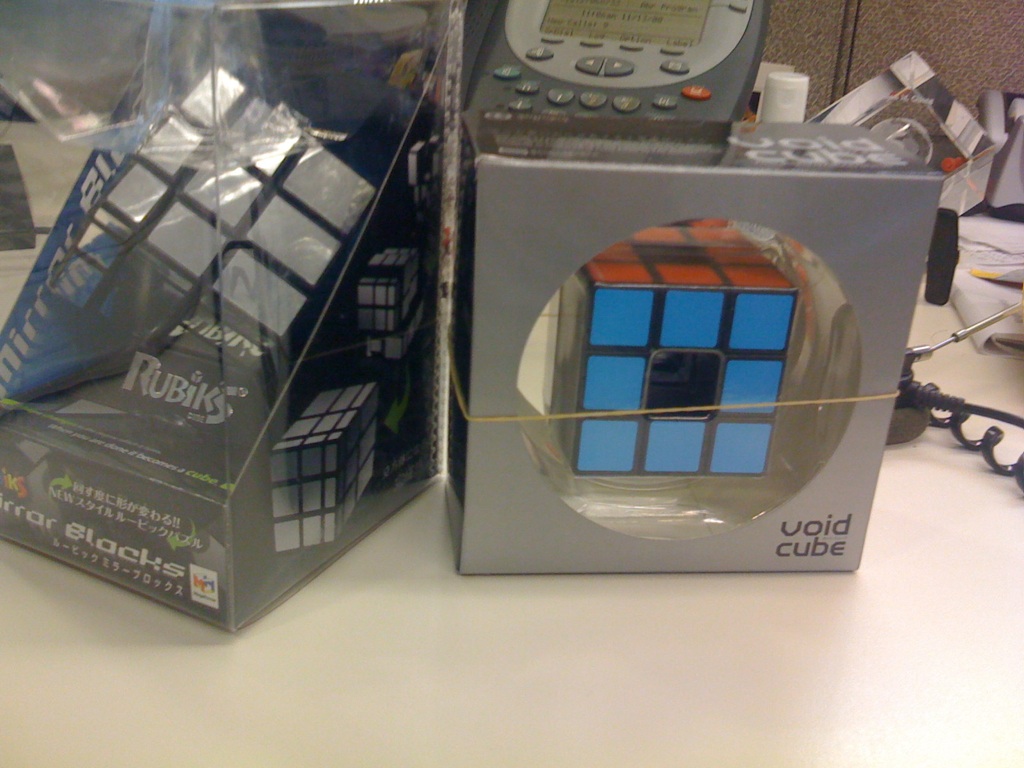The image depicts a void cube still sealed in its original packaging, prominently displayed on a desk. The void cube, similar in appearance to a traditional Rubik's cube, features blue and red faces. Unlike a standard Rubik's cube, the packaging specifically labels it as a "Void Cube." Unique to the blue section of the cube, there is an additional black square at its center. The package is secured with a rubber band. To the left of the void cube, another packaging houses a traditional Rubik's cube, distinguishable by its silver color and marked with the "Rubik's" branding. The backdrop reveals an office telephone, along with assorted notes and papers, adding to the everyday work environment setting. The entire scene is well-illuminated, presenting a bright and clear image, emphasizing the vividness of the items displayed.